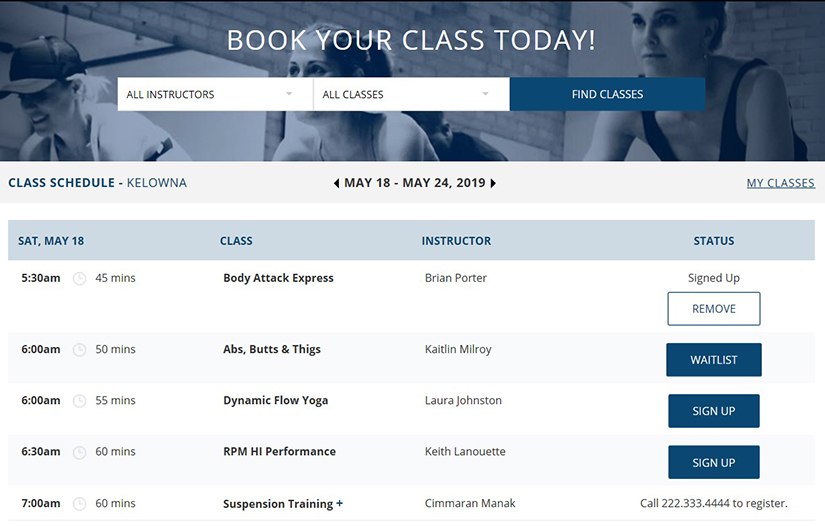This detailed screenshot of a website displays a booking interface for fitness classes. At the top, the phrase "Book Your Class Today" is prominently shown in white text. Situated directly below are selection menus with drop-down options. On the left, users can filter by "All Instructors," while the middle section includes a filter for "All Classes." The right side features a "Find Classes" button, enabling users to search for specific classes by type and instructor.

In the top left corner, the text "Class Schedule" clarifies the current view is for Kelowna. Centered at the top is the date range "May 18th - May 24th, 2019," indicating the week’s schedule. The top right corner contains a "My Classes" section, showing classes that the user is either enrolled in or waitlisted for.

The detailed schedule includes:
- **Saturday, May 18th at 5:30 a.m.**: A 45-minute "Body Attack Express" class with instructor Brian Porter, for which the user is signed up.
- Another class titled **"Abs, Butts, and Thighs"** is scheduled for 50 minutes with instructor Caitlin Milroy. The user is waitlisted for this class.
- The user is waitlisted for all other classes in the displayed schedule.

This user interface allows seamless booking and tracking of fitness classes by offering clear options for filtering, scheduling, and viewing class enrollments and waitlists.